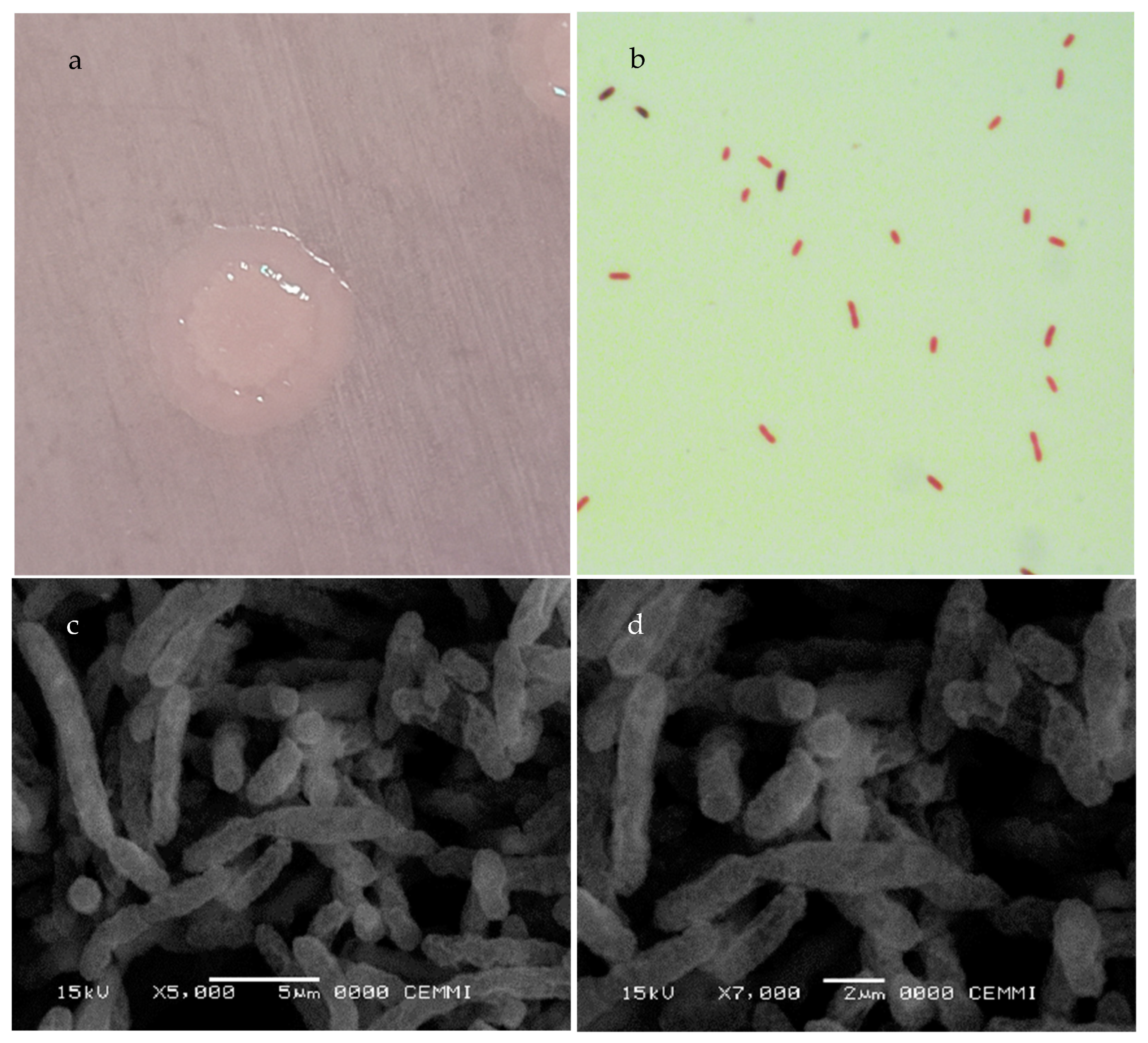This image features an array of four labeled photos, each providing a detailed microscopic view. The labels, in black ink, identify the images as A, B, C, and D starting from the top left. 

In Photo A, located at the top left, there’s a close-up view of a surface showcasing a shiny, pinkish, circular substance that resembles melted wax or a spill. This appears to be an off-white droplet on a whitish background.

Photo B, at the top right, presents a microscopic view of numerous narrow, cigar-shaped objects that are reddish in color set against a very light green background. These objects—possibly microorganisms—number a couple of dozen and are arrayed in various orientations.

Photo C, on the bottom left, offers a 5,000x magnified, black-and-white image of a dense collection of elongated objects that could be microorganisms similar to those seen in Photo B. These objects are in a mix of white and dark hues with black spaces between them, resembling a tangled mass of spaghetti. The bottom of this image includes white text indicating "15 kV," magnification "X5,000," and a length scale "5 µm."

Photo D, at the bottom right, shares similarities with Photo C but features a less dense collection and higher magnification. The 7,000x magnified image shows these cigar-shaped organisms in greater detail, emphasizing their distinct outer layers. The bottom text reads "15 kV," magnification "X7,000," and a length scale "2 µm," along with the text "CEMMI."

Overall, the series provides intricate views of what seem to be various microorganisms under increasing magnifications, with clear annotations on scale and magnification.